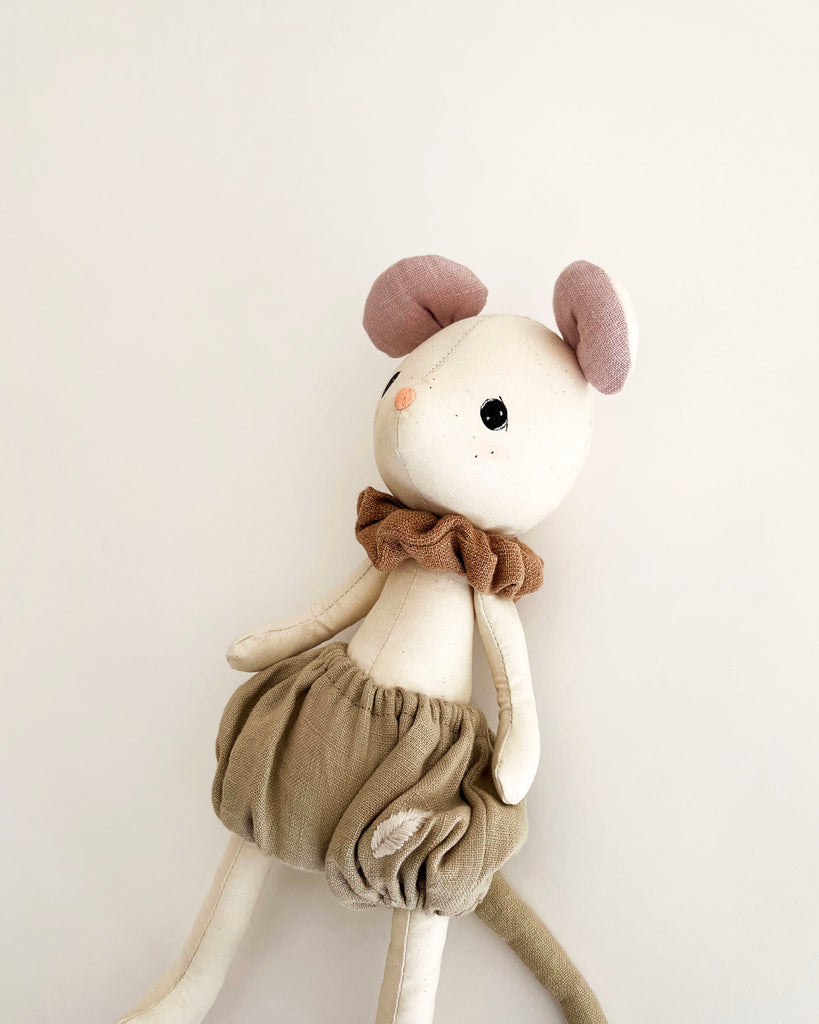The image depicts a handmade stuffed doll of a light beige mouse, characterized by its anthropomorphic features and cutesy appearance. The mouse has large, dark eyes that give it a calm expression, a little pink nose at the tip of its snout, and small pink ears atop its head. It is dressed in textured, burlap-like bloomers that resemble poofy shorts or bell-bottoms, with its hairless tail also covered in the same fabric. Around its neck, the mouse wears a brown collar that looks like a small scrunchie. The doll is positioned looking toward the left against a neutral white or very light-colored background, allowing the details of the doll to stand out starkly.